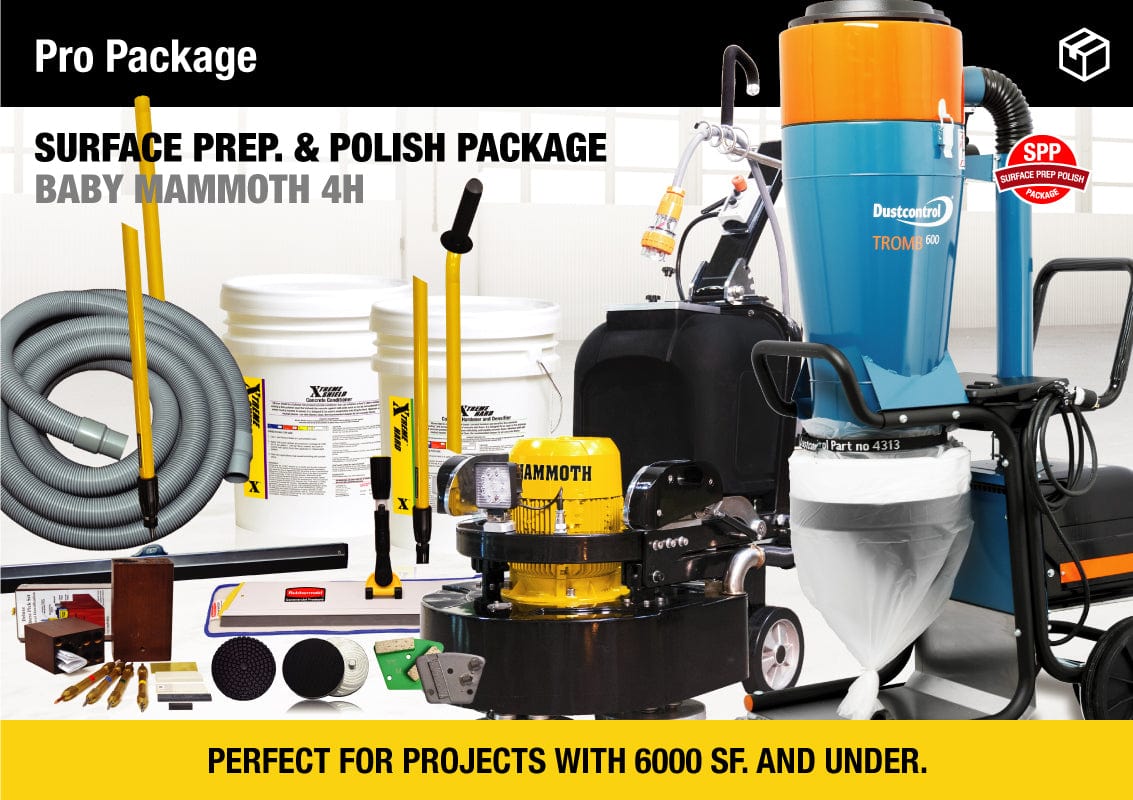This advertisement showcases the ProPackage Surface Prep and Polish Package, Baby Mammoth 4H, ideal for projects up to 6,000 square feet. Dominating the center is a large, black and yellow device labeled DustControl TROMB, which suggests capabilities similar to industrial vacuums or floor polishers; the yellow canister bears the Mammoth branding. The top-left corner features white text reading "ProPackage," with black text below spelling "Surface Prep and Polish Package" and gray text indicating "Baby Mammoth 4H." Accompanying the main device are various cleaning and surface prep tools, including a gray hose, attachments with yellow and black handles, and several mysterious black circles. The advertisement also includes other industrial-sized apparatuses like buckets, hoses, and possibly mops or waxers, highlighting their application in large-scale cleaning or floor refinishing projects. A yellow banner at the bottom emphasizes its suitability for areas under 6,000 square feet. Additional branding elements include a red circle logo with "SPP" and an unreadable small text, along with a white logo depicting a boxed item with packing tape.